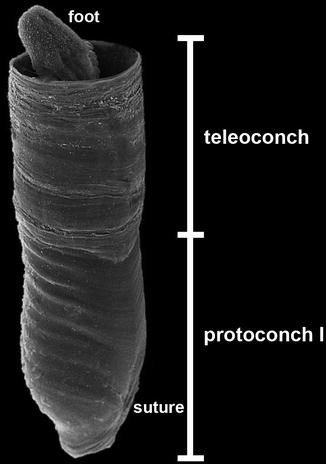The black and white image appears to be taken with an electron microscope and depicts a close-up of a microscopic creature. The creature exhibits a shapeless, oblong structure resembling a sock, with a smaller protrusion at the top labeled "foot." The central structure is segmented and annotated with labels; "teleoconch" at the upper half, "protoconch" at the lower half, and a vertical "suture" line running down its length. The background is solid black, while the segmented body of the creature appears in varying shades of dark gray and white, with a textured surface suggesting it is not smooth. The clear, bold white text labeling the parts stands out distinctly against the stark background, making the annotations easily readable.